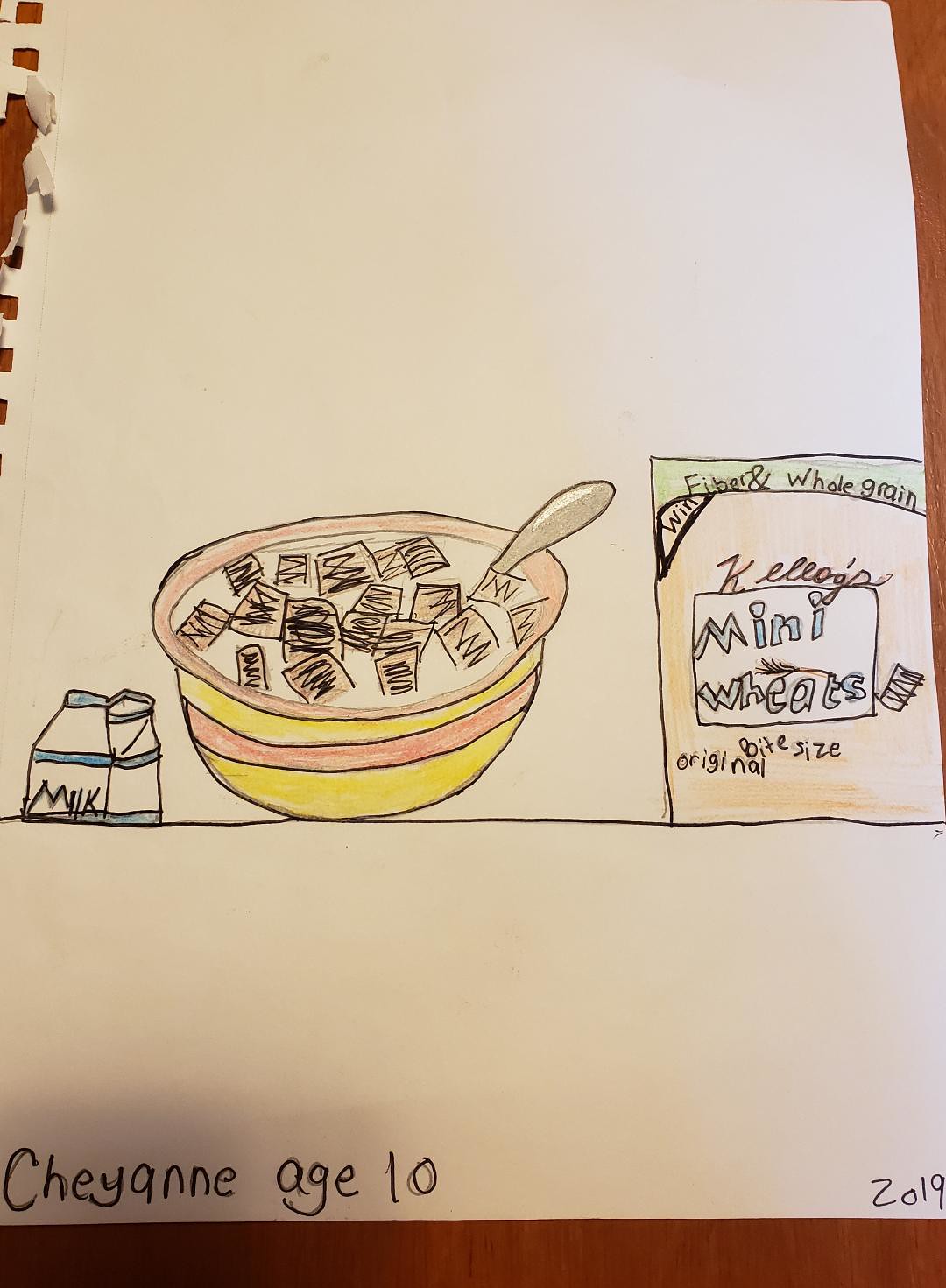This image, drawn by a child named Cheyenne at age 10 in 2019, is meticulously detailed on a plain white sheet of paper and depicts a breakfast scene on a wooden table. To the left side of the image, there is a squat, short milk carton colored white with blue stripes. The word "milk" is written on it in black. In the center, there is a yellow bowl with an orangey-red stripe and an orange rim, filled with cereal, white milk, and black scribbles representing the cereal pieces. A silver spoon rests inside the bowl. Additionally, there is a cereal box on the right side, labeled at the top in black against a green background with "fiber whole grain." Below, in black font, it reads "Kellogg's," followed by "mini-wheats" in blue font. An illustrated cereal piece is present on the box, and the phrase "original bite size" appears in black font. The entire scene is carefully arranged on a wooden table, capturing a classic breakfast setup.